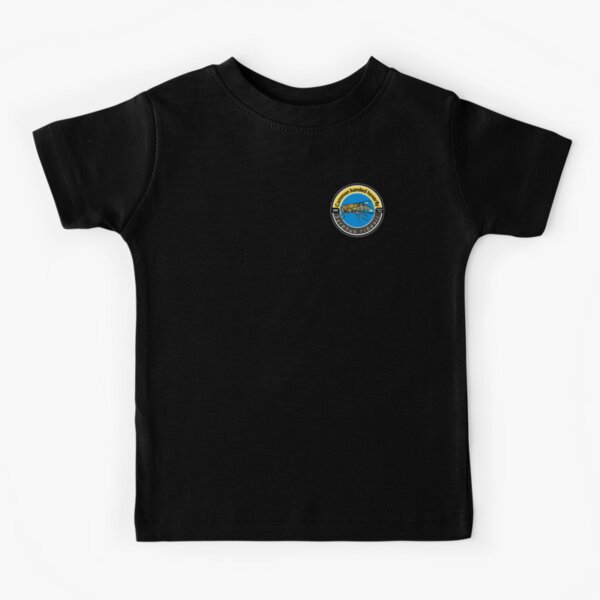This image features a black crew neck t-shirt with short sleeves, meticulously ironed to remove all wrinkles. Positioned against a grey background, the t-shirt prominently displays a small, intricate logo on the left breast area. The logo is circular with a yellow top arch and a grey bottom arch, enclosing a blue inner circle. Within the blue circle, there is an image resembling a bee or wasp with its body centrally placed, head facing left, and wings near its tail. Although the text within the logo is present, it is too small to read clearly.